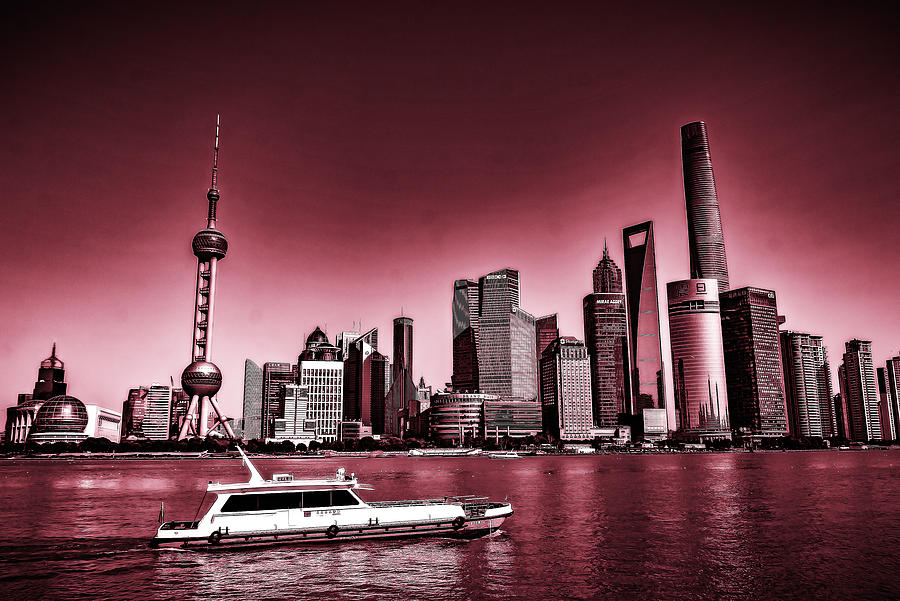This image is an artistically composed illustration of a city skyline, imbued with a dramatic red-to-magenta gradient that gives it an otherworldly atmosphere. The foreground features a body of water with subtle ripples, on which a white boat with black tinted windows is sailing from left to right, positioned centrally. The skyline in the background is densely packed with skyscrapers and rectangular buildings with numerous windows and dozens of floors. Notable among these structures is a tall, slender building reminiscent of the Space Needle on the right, and another rectangular building with a distinctive rectangular hole at the top. The sky above the city is filled with a scattering of stars, adding to the surreal quality of the scene. The entire composition is bathed in hues of red, mahogany, and magenta, creating a captivating and somewhat eerie visual effect.